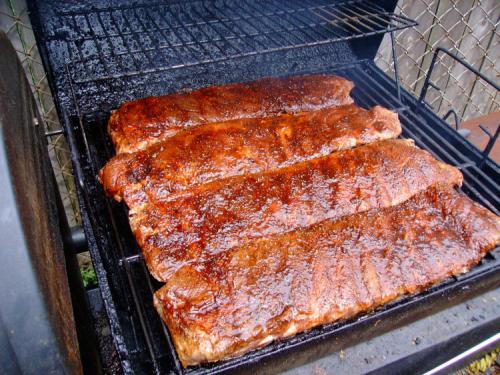This close-up photograph showcases barbecued spare ribs cooking on a worn-out, filthy grill. The ribs, slathered in barbecue sauce, are charred and crusted, making it challenging to definitively identify the type of meat. However, their slightly delicious appearance manages to shine through despite the grill's neglected state, which is visible on its side and base, scattered with charcoal and ash debris. No identifiable time or date stamps the image. To the right, a chain link fence partially comes into view, adding a gritty context to the scene. The overall impression is of a makeshift smoking or grilling setup, capturing a gritty yet appetizing glimpse of the barbecuing process.